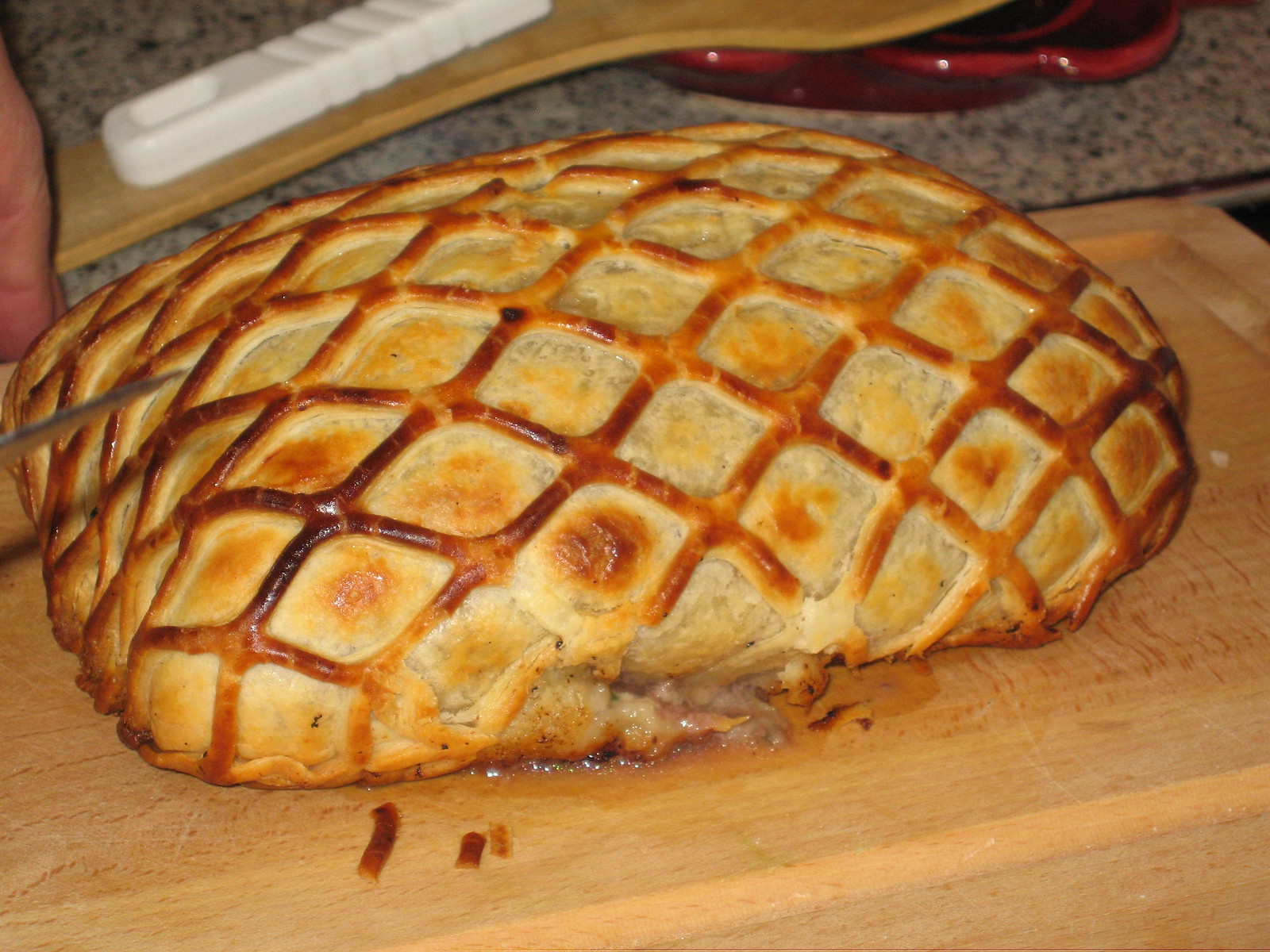In this image, we see a round loaf of bread with an intricate checkered pattern on its golden-brown crust, suggesting it has been baked to perfection. The squares are bordered in dark brown, with slightly burnt white and yellow centers on most of the top surface, creating a visually appealing texture. The bread appears to be resting on a wooden cutting board, with various kitchen utensils placed above it, indicating a kitchen setting. Sticking out subtly from underneath the loaf is a brown element, possibly a portion of meat or a bird's wing, adding an element of mystery to the dish. A person stands behind the board, poised to cut the loaf with a knife, contributing a sense of anticipation and human presence to the scene. The background reveals a kitchen countertop with some visible cooking utensils, completing the domestic atmosphere of this culinary scene.